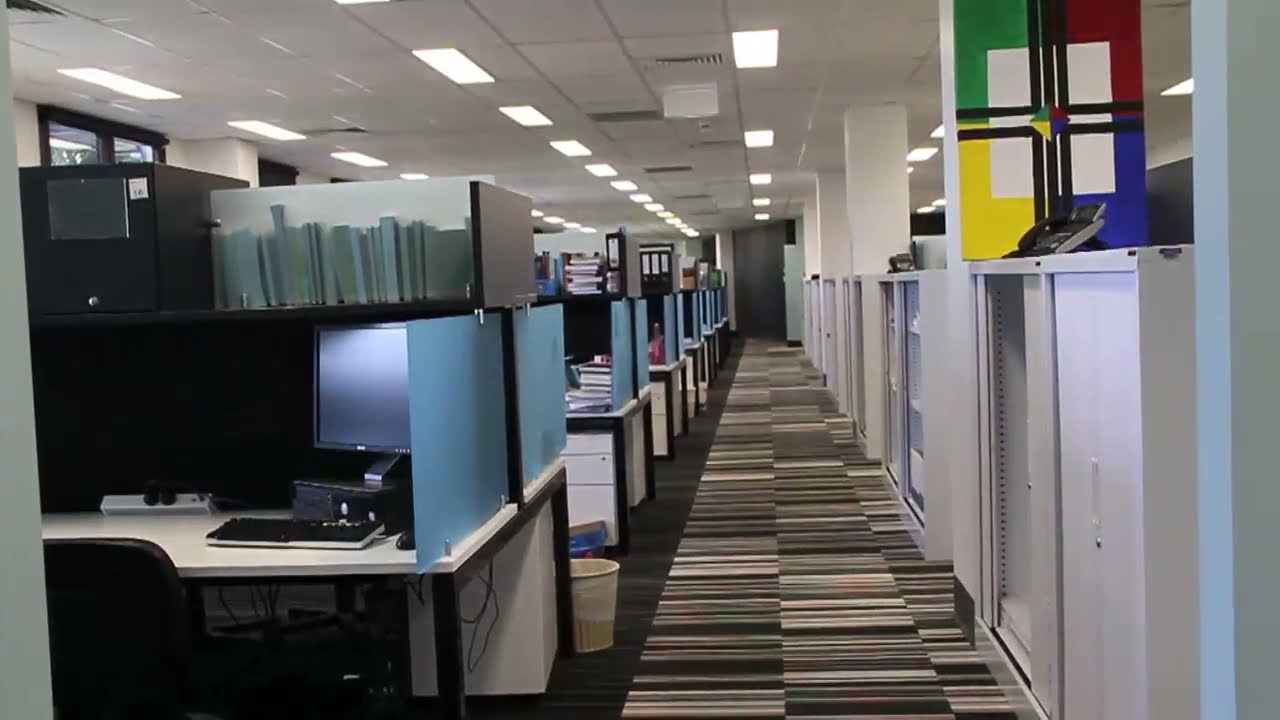The image is a horizontal rectangular box showcasing the side of a large, light and dark tan building, presumed to be in a public or academic setting. The building's facade features about six to eight dark-colored windows arranged along the top, likely the second floor, and other windows along the bottom, presumably on the ground floor. On the left side of the image, a tall tree extends nearly to the top and cuts off at the bottom. To the right of the tree, slightly off-center, there's a doorway with some illegible lettering above it, possibly saying "Human Resource Building." At the bottom, the entry doors are visible.

In the lower right, a tree limb with red flowers protrudes into the frame. Black street lamps are present in the scene, adding to the frame's detail. Superimposed over the middle of the image in white letters are the words "Tourism Policy and Planning," suggesting that this image might be part of a presentation, possibly about a company's offerings related to tourism. The overall tone of the image is darker, almost as if it’s slightly faded, contrasting with the white highlighted text that draws the viewer's attention.